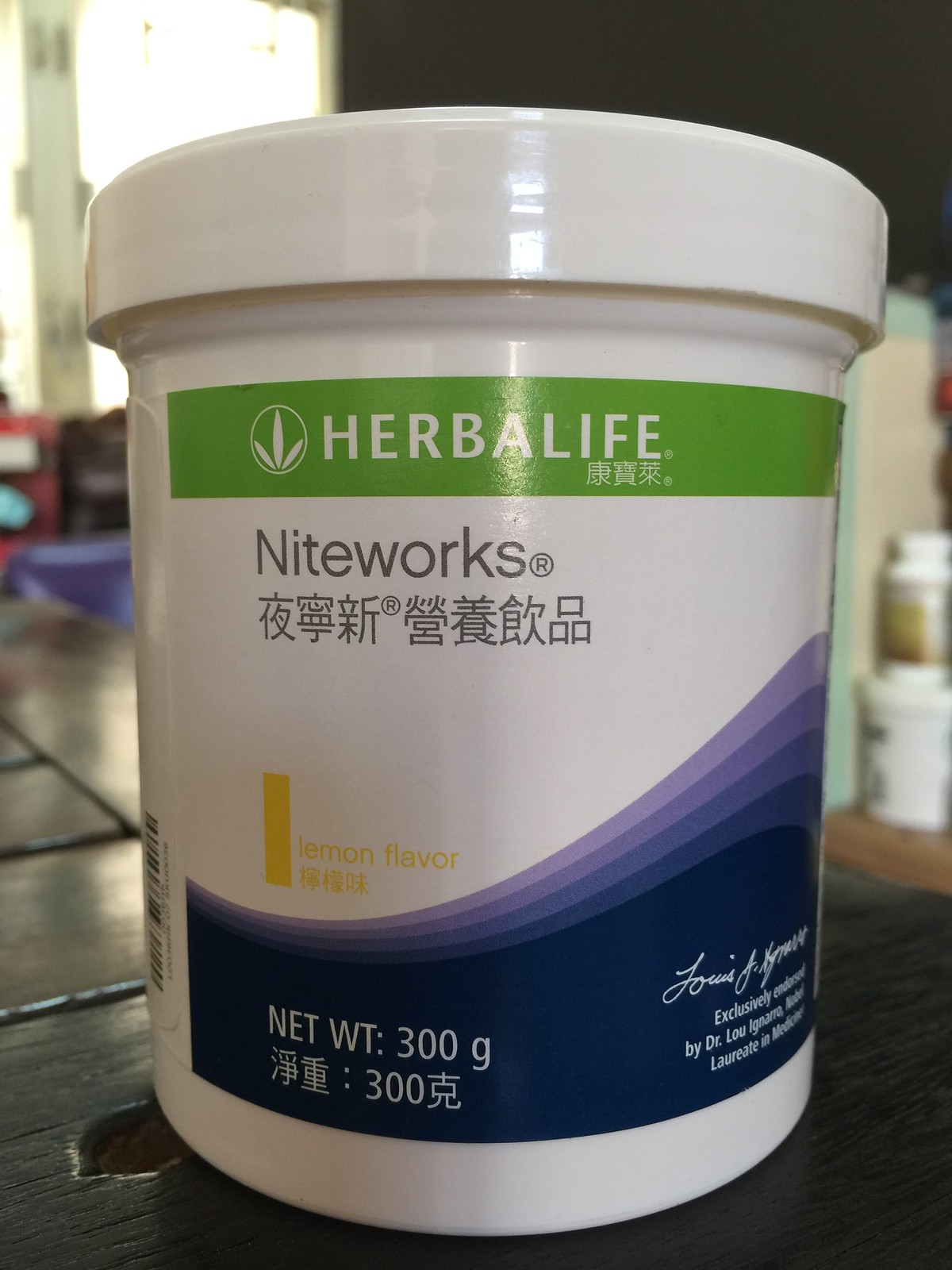This is an up-close photograph of an Herbalife supplement container. The container is white plastic with a screw-on top and features a detailed label. At the top of the label, a green banner displays the word "Herbalife" in white print. Beneath the green bar, the product name "Nightworks" appears in black lettering alongside a row of Asian characters. Toward the bottom left of the label, a yellow bar announces "Lemon Flavor." Lower down, a multicolored wave pattern in shades of blue and purple highlights "Net Weight 300 grams" and more text in Asian characters. The bottom right corner features the signature "Exclusively by Dr. Lu." The container sits on a surface that appears to be either ceramic black tile or a wood-like counter, accompanied by a small water spill to the left. In the background, several white jars of vitamins or other supplements are visible, one with a gold label.